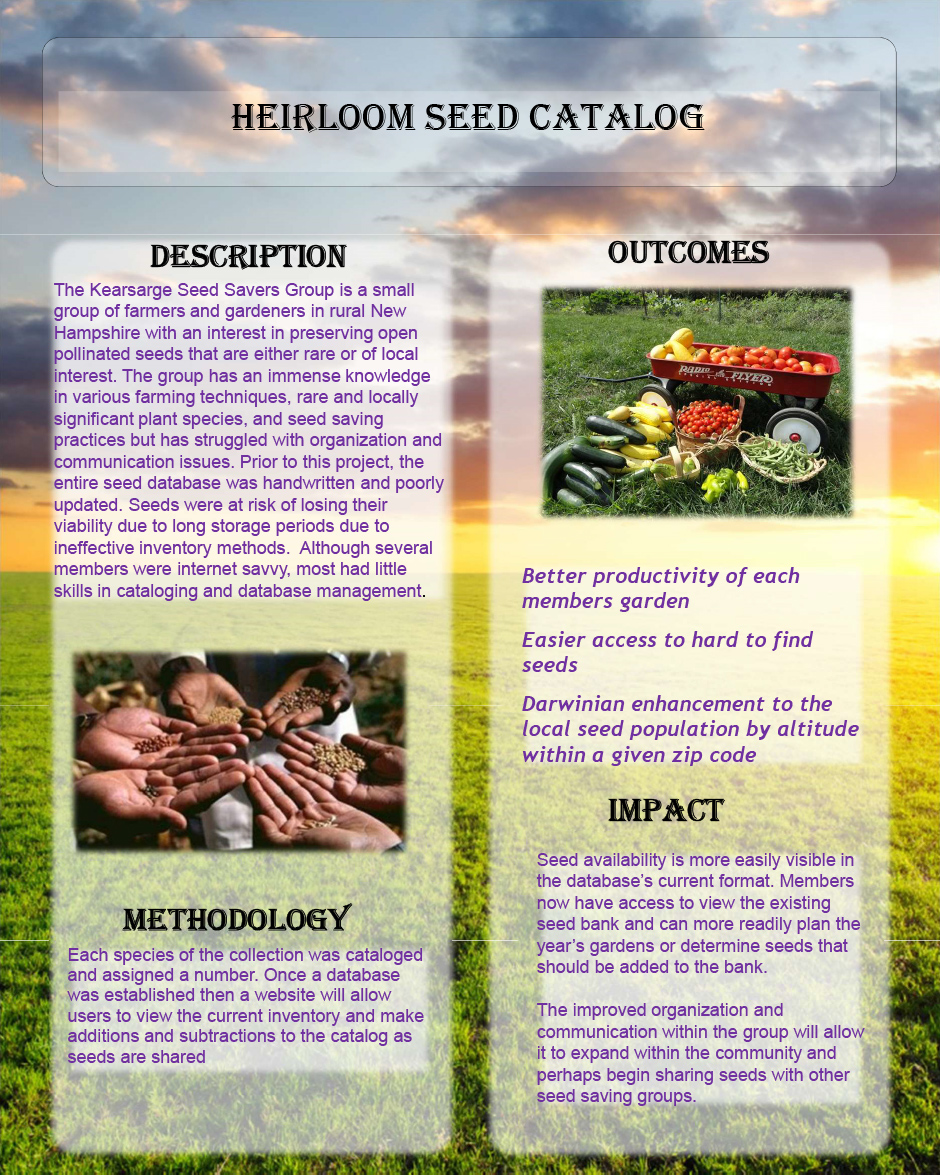The image is an intricately detailed page from an heirloom seed catalog. The upper part of the image showcases a picturesque sky with blue hues, gray clouds, and sunlight breaking through, reflecting beautifully on the scene. The background features a lush field of grasses, bathed in warm sunlight, creating a serene countryside atmosphere. 

At the top center of the page, the label "Heirloom Seed Catalog" is prominently displayed in black text. The page is divided into several sections with the following headings: "Description," "Methodology," "Outcomes," and "Impact," each accompanied by detailed paragraphs.

In the "Description" section, located in the upper left corner, the text details the Kearsarge Seed Savers Group, a small collective of farmers and gardeners in rural New Hampshire who are passionate about preserving rare and locally significant open-pollinated seeds.

On the upper right corner, under the "Outcomes" heading, there is an image of a Radio Flyer red wagon filled with a bountiful harvest of tomatoes, cucumbers, and other garden vegetables, resting on a grassy field.

The bottom left features a powerful visual of diverse hands holding a variety of valuable seeds, symbolizing the preservation efforts. Meanwhile, the "Methodology" section occupies the lower part of the page, explaining the processes involved in seed preservation. The "Impact" section in the bottom right corner further elaborates on the significant effects and benefits of their preservation activities.

Overall, the page offers an appealing blend of visual and textual elements, capturing the essence of heirloom seed preservation and the dedication of the Kearsarge Seed Savers Group.